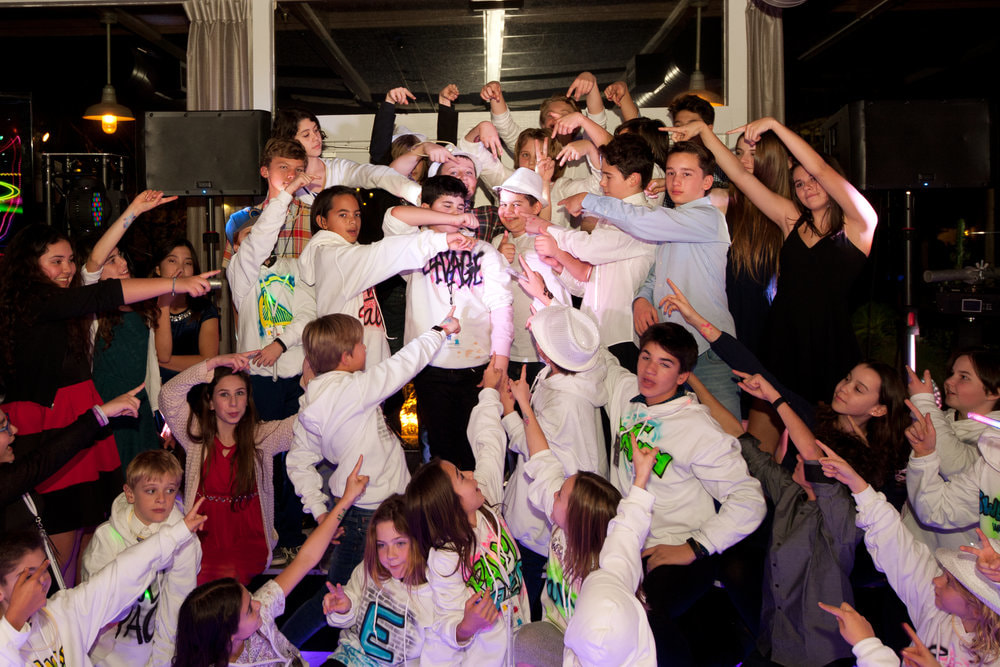This color photograph captures a lively scene of approximately 30 teenagers gathered indoors, likely in a venue with a stage and arcade games faintly visible in the dimly lit background. Most of the teens, a mix of boys and girls, are joyfully pointing towards the center where a smiling young man stands out, wearing a white fedora and flashing a thumbs up. The group is predominantly dressed in white hoodies adorned with bright, hand-drawn-style graffiti, though some wear regular street clothes. Adding to the playful atmosphere, one person near the central figure is holding up a peace sign next to his head. The backdrop features curtains, a speaker to the left, and a possible arcade machine, enhancing the sense of a fun, communal gathering. Despite varying expressions, from distracted to exuberantly happy, the overall mood is one of camaraderie and celebration.